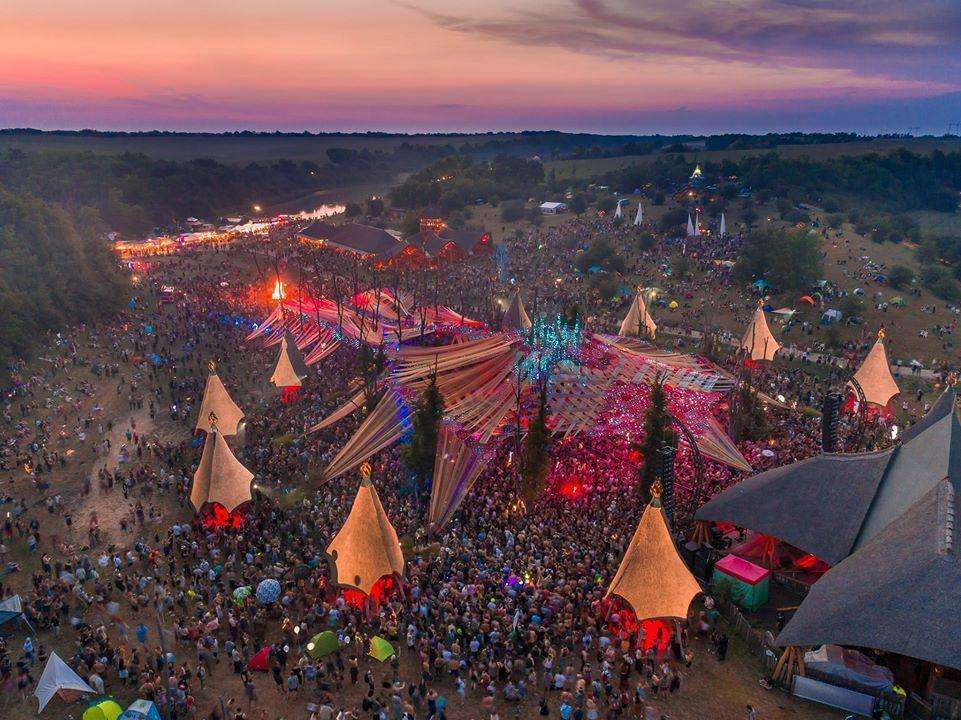The aerial photograph captures a vibrant festival against the backdrop of a stunning early evening sky, painted in a blend of coral, pink, purple, and blue hues with feathery gray clouds in the upper right corner. The event is held on a predominantly dirt-covered ground with patches of green grass, flanked by trees on the upper left and rolling hills on the upper right. Dominating the center of the image is a large, multicolored tent illuminated by blue, pink, yellow, and brighter blue lights, casting a magical ambiance. Surrounding it are numerous smaller, tan triangular tents and large tan umbrellas with red undersides, creating a sprawling labyrinth of canopies. Thousands of people are densely packed around the central tent while many others are scattered throughout the scene, even extending to a treelined area in the upper right background and a river with light-reflecting black-topped tents along the left side. The festival atmosphere is further enhanced by golden lights, contributing to the bright and celebratory mood of the gathering.